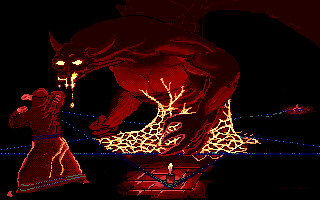A small, vibrant cartoon image features a dominant, colossal red dragon with black patches along its back and rear end. The dragon's fierce white eyes and dripping white liquid from its mouth create an intimidating presence. Its red ears stand out prominently. In the flaming red and blue background, another character—also in hues of blue and red—is depicted gazing upwards. This character appears to be looking at a lion-like creature with striking pink eyes and a pink mane around its neck. Additionally, in the corner of the image, a tiny person is seen observing the scene, adding a touch of perspective to the fantastical depiction.